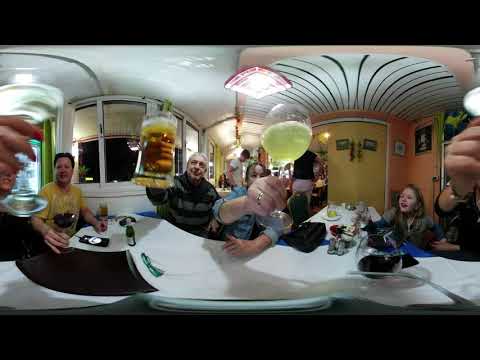This panoramic photograph features a festive scene of multiple people gathered around a rectangular table with several chairs. The backdrop includes walls painted in vibrant hues of yellow and orange, and a white ceiling adorned with black stripes. A large multi-pane window with a yellow pull-down curtain is prominently situated next to the table, set within a white window frame. The attendees, which include an older man, a woman with short hair, a young woman in a blue denim shirt with rolled-up sleeves, and a child, are raising various glasses in a celebratory toast. The man in a black and gray striped hoodie holds a beer stein filled with amber liquid, and the woman in the denim shirt has a wine glass with a yellow liquid. The setting, possibly a restaurant or a dining room, exudes a joyful, celebratory atmosphere. The white ceiling features black lines resembling a clamshell pattern and includes a square light, adding a unique design element to the room.